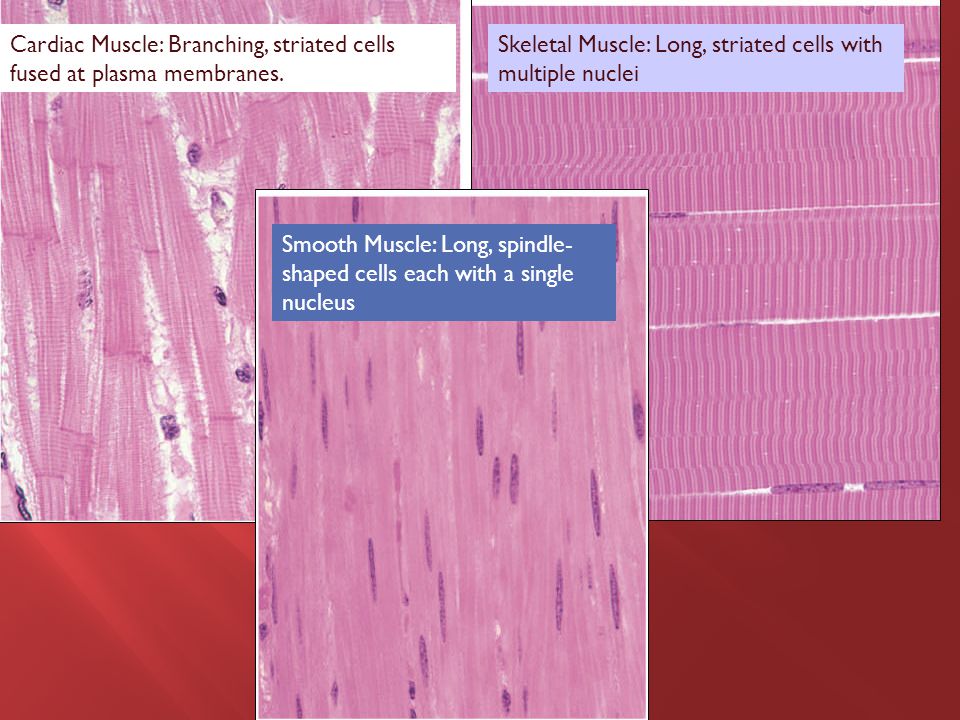The image is a detailed illustration, likely intended for an informational pamphlet or medical poster, showcasing three types of muscle tissue against a rich maroon and red background interspersed with pink and purple hues. In the top left corner, a white rectangle holds the text “cardiac muscle: branching striated cells fused at plasma membranes,” overlaid on an image of cardiac muscle tissue, depicted in pink with white interspersed. To the right, a lavender rectangle contains the words “skeletal muscle: long striated cells with multiple nuclei,” overlaying an image of skeletal muscle tissue arranged in vertical, pink-hued brush strokes. Centrally positioned is a blue rectangle that reads “smooth muscle: long spindle-shaped cells, each with a single nucleus,” superimposed on an illustration of smooth muscle tissue showcasing elongated spindle-shaped cells in a pink shade. The colors and overlapping panels create a visually cohesive educational tool for a medical setting.